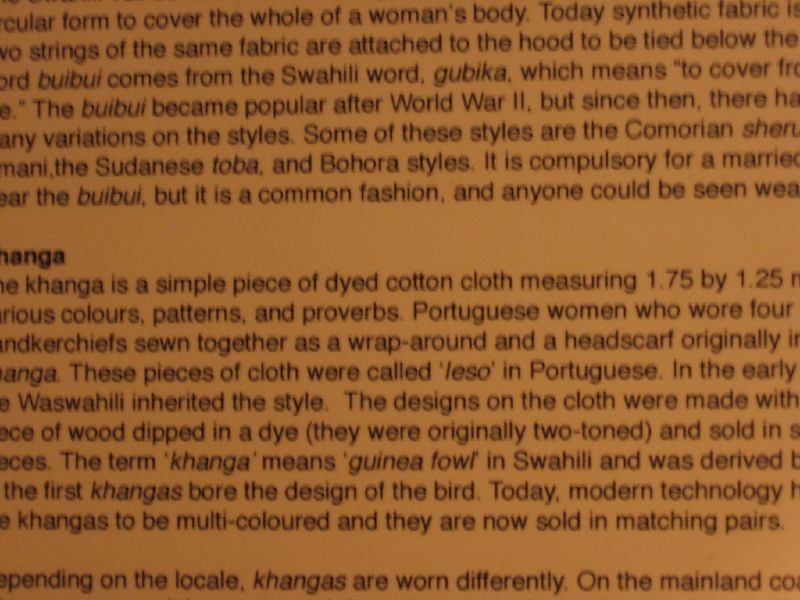The image showcases a zoomed-in photograph or scan of a brown book page filled with a text divided into three paragraphs. The text is typed and appears to discuss traditional garments with some of the words extending beyond the edge of the image, making them partially cut off. The first paragraph explains that the "bwibwi" is formed to cover the whole of a woman's body using synthetic fabric, and that strings of the same fabric are attached to a hood to be tied below. The term "bwibwi" originates from the Swahili word "gubika," which means "to cover." The bwibwi became popular after World War II, but numerous variations now exist, including the Camorian, Sudanese toba, and Bohora styles. While it is compulsory for married women to wear the bwibwi, it has become a common fashion, and anyone can wear it.

The second paragraph shifts focus to the "kanga," described as a simple, dyed cotton cloth measuring approximately 1.75 by 1.25 meters. Traditional kanga designs include various colors, patterns, and proverbs. Initially, women in Portuguese communities wore pieces of cloth known as "leço," which were sewn together as a wraparound and headscarf. The Swahili later inherited this style. Originally, kanga designs were created using wood dipped in dye, featuring two-toned patterns and were sold with designs depicting the guinea fowl, from which the term "kanga" is derived. Today, with the help of modern technology, kangas are multicolored and sold in matching pairs.

The final visible line notes that depending on the locale, kangas are worn differently on the mainland, suggesting regional variations in the style and method of wearing the kanga.